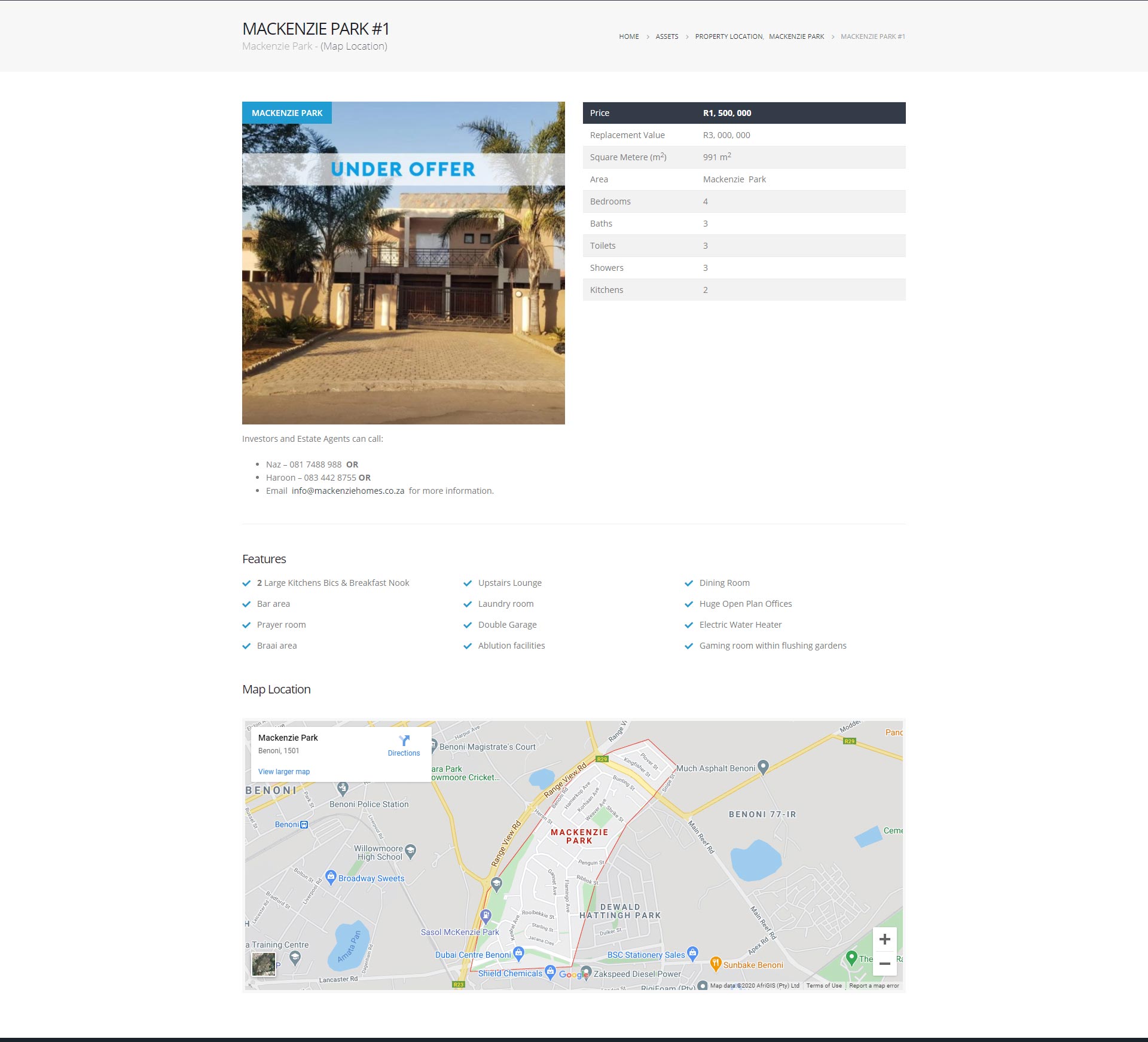**Detailed Caption:**

The image showcases a detailed webpage for a real estate listing in Mackenzie Park. The top of the page prominently displays the title "Mackenzie Park No. 1" along with a location map of Mackenzie Park. The webpage is structured with various sections including Home, Assets, Property Location, and another instance of Mackenzie Park, emphasizing the property's prominence.

Central to the page is a high-quality image labeled "Under Offer," depicting a charming home featuring a gate, multiple palm trees, a driveway, and lush landscaping. The property is listed with a sale price of R1,500,000 and a replacement value of R3,000,000. The home boasts a substantial area of 991 square meters and is located in the scenic area of Mackenzie Park.

Detailed property specifications include:
- Four bedrooms
- Three bathrooms
- Three toilets
- Three showers
- Two kitchens

Additionally, the listing provides further features and amenities such as:
- Two large kitchens equipped with a fixed breakfast nook
- A cozy bar area
- A designated prayer room
- A spacious upstairs lounge
- A functional laundry room
- A double garage
- Comprehensive ablution facilities
- A formal dining room
- Expansive open-plan offices
- An electric water heater
- A gaming room with beautifully maintained gardens

Investors and estate agents are encouraged to contact via the provided phone number D817488988 or email info@MackenzieHomes.co.za for more details. The page also highlights the exact location of the property within Mackenzie Park on a map. The overall design of the webpage features a clean white background, interspersed with various illustrative images.